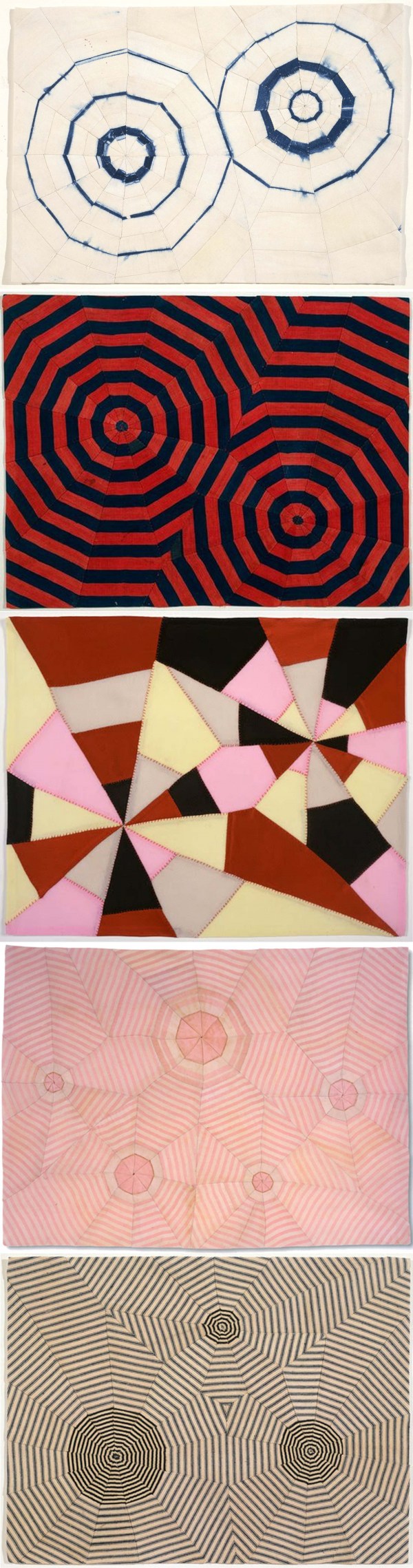This abstract artwork is a vertical composite consisting of five seamless rectangular panels of equal dimensions. The top panel features a beige background with two juxtaposed cells, each containing a nucleus and cell wall—one cell is notably larger than the other. Below it, the second panel displays concentric circles in vibrant red and black hues, creating a hypnotic pattern that progresses from small to large. The third panel showcases an intricate mosaic of overlapping triangles in shades of pink, yellow, beige, and gray. The fourth panel has a pink backdrop highlighted by a centrally placed circular section, accentuated with delicate lines and additional circles. Finally, the bottom panel presents three circles of varying sizes (a large one on the left, a medium one on the right, and a smaller one on top) arranged in a triangular formation. Surrounding these gray blobs are rhythmically drawn concentric lines that resemble a spiderweb, rendered in black. The entire image lacks any textual information, making the visual elements the sole focus.